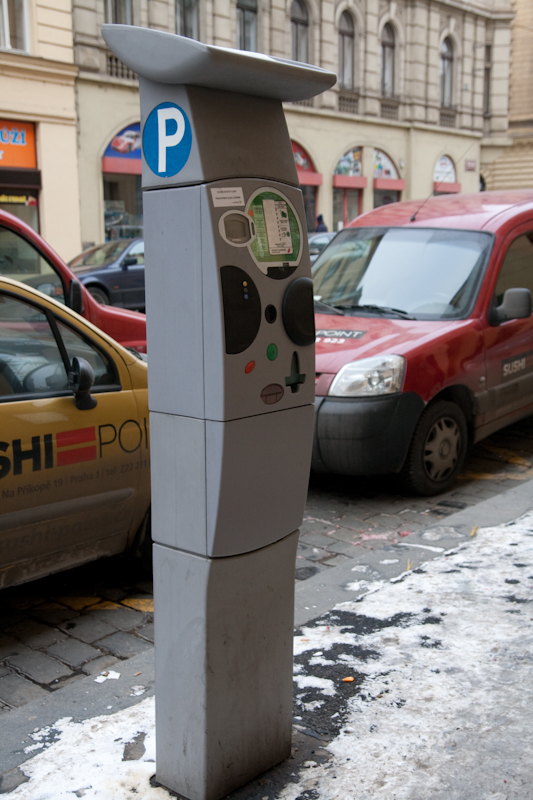This color photograph depicts a bustling city street, dominated by a parking meter, which features a gray post with a blue circle and a white "P" indicating parking. The parking meter has an interface with a screen likely used for selecting parking time, a slot for debit cards, and red and green buttons for transaction processes. Flanking the buttons are two black circular elements. Behind the parking meter, a yellow vehicle with black writing, possibly a taxi or police car, is parked, displaying two reddish lines akin to an equal sign. In front of it is a red compact transit van. The background reveals the street's other side, showcasing an old 19th-century building with arched windows and a stone facade, indicating storefronts on the ground level and more detailed stone brickwork on the upper levels. A blue car is also visible on that side of the street.